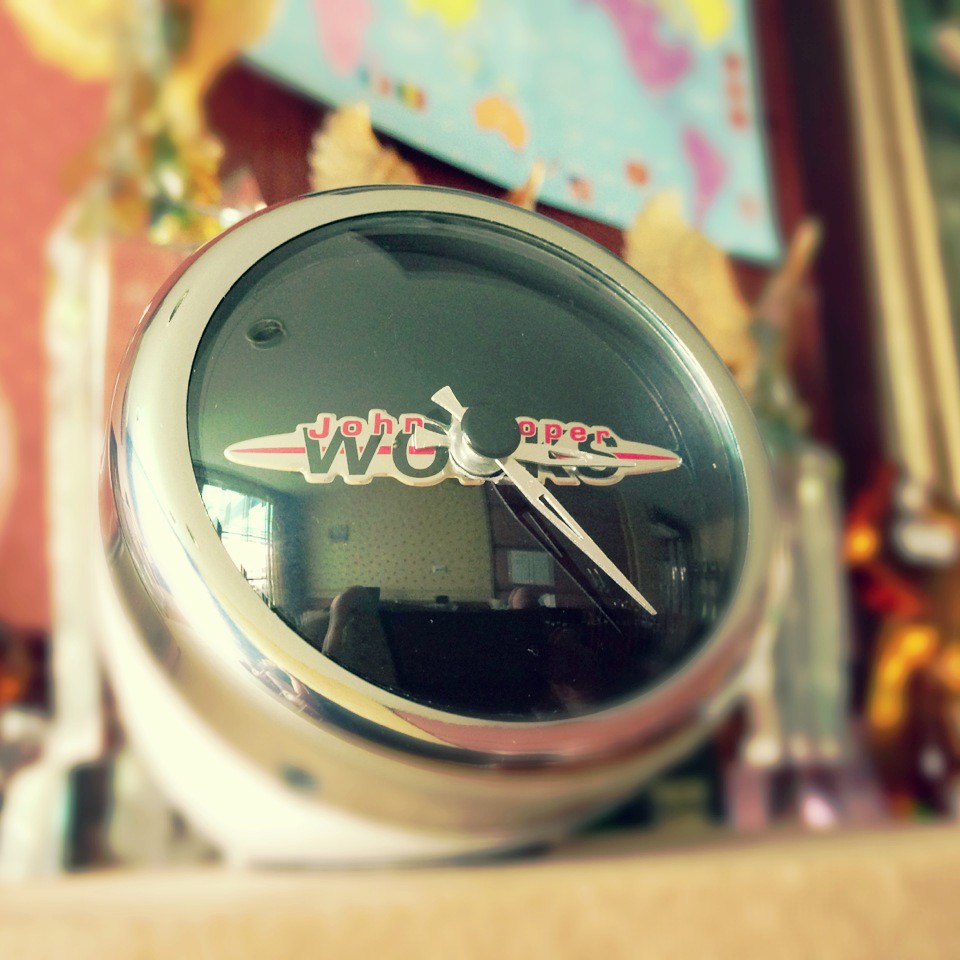The image features a distinctive clock placed on a shelf. The clock has a green face with bold red letters outlined in white, spelling out "John Oper". Below this, the word "works" is displayed in green letters on a white background with a red stripe running through it, creating the phrase "John Operworks". The white background forms a wing-like design with the red stripe cutting across it. Positioned at the center of the clock is a green button, around which the white minute and second hands are set, currently showing the time as approximately 3:25. The clock is framed by a gold band, adding a touch of elegance, and the back of the case is white, giving it a deep-set appearance. The shelf on which the clock sits is also adorned with trophies and a partially visible map, though these background details are somewhat out of focus, drawing attention to the intricately designed clock.